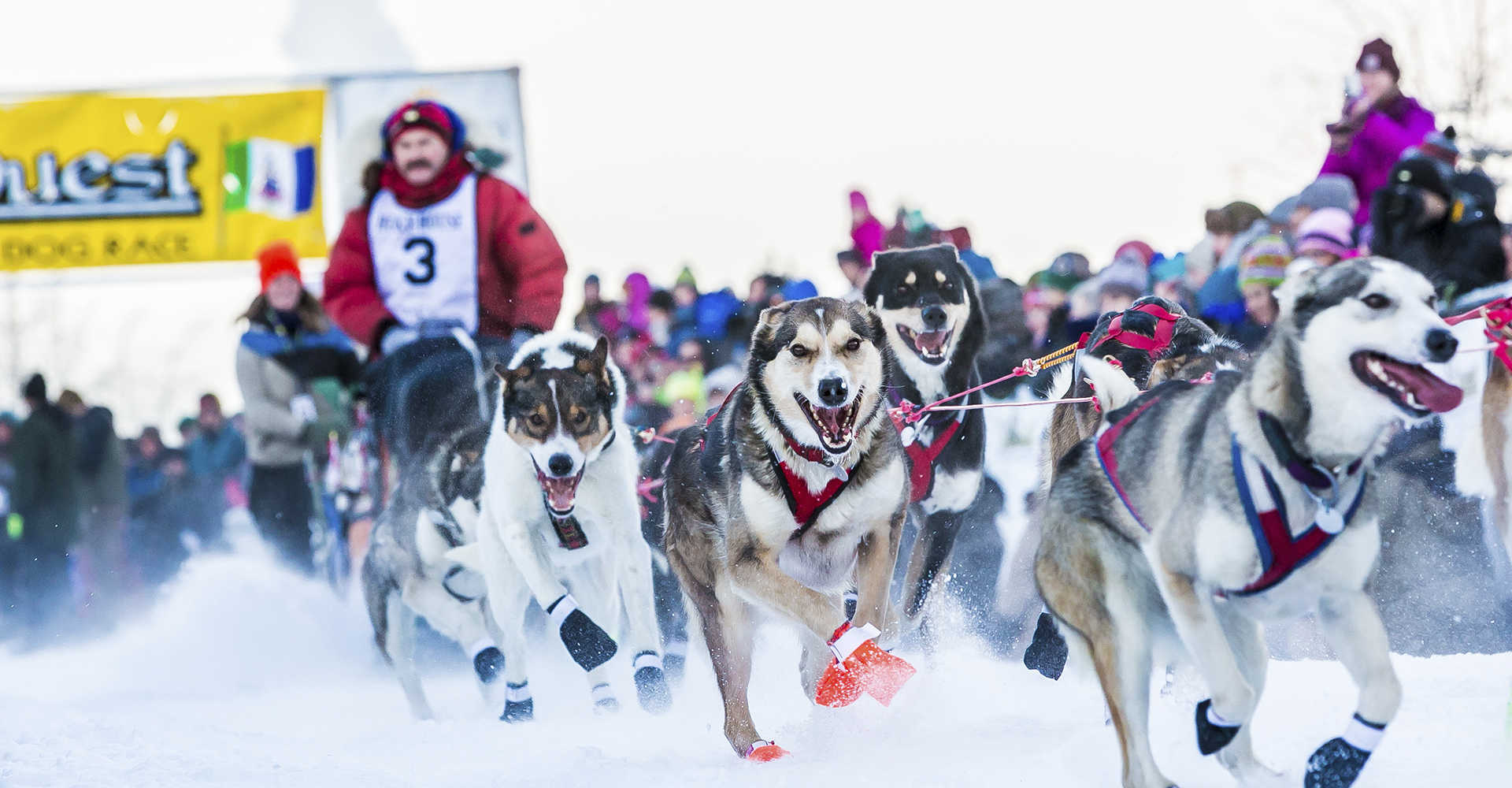In this professionally captured image, we see the intense start of a dog sled race set in an expansive snowy landscape beneath a white, cloudy sky. In the foreground, a team of energetic huskies, mostly grayish-white and black, all wearing blue snow shoes, are captured in full motion with no motion blur, emphasizing their dynamic movement as they pull the sled. Leading from the sled is a musher clad in a red puffy coat, red scarf, and hat, and his vest prominently displays the number three in white. Behind the team, the scene softens into the background, where a vibrant yellow banner with white, green, and blue flag details marks the finish line. The right side of the image features a crowd of spectators and media members, all intently watching and documenting the race as it unfolds.